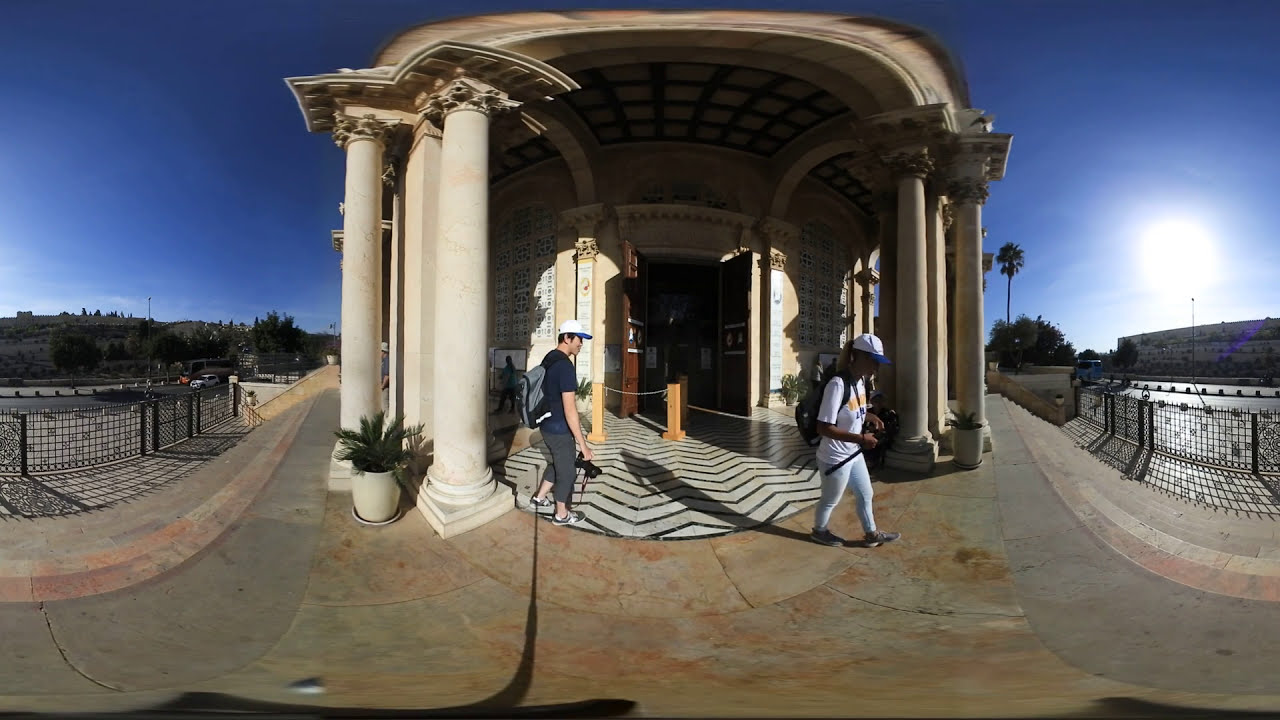The image captures a stucco, white stone building centrally positioned under a wide-angle lens, causing notable curved distortion. Prominent columns line the front of the building, flanked by two large, open brown doors. Two individuals, a man on the left and a woman on the right, are engaged in activity near the entrance—one appears to be exiting while the other is entering. A palm tree is situated near the columns enhancing the tropical atmosphere.

The surrounding scene includes an orange marbled terra-cotta pavement that stretches wide, with shadows cast by both the building and a black, gridded metal fence. The low sun on the right side contributes to elongated shadows, casting dramatic patterns across the pavement. In the background on the left side, a tree-lined hill contrasts against a blue sky, adding depth to the image, while railings and fences on the periphery, also subject to the lens-induced warp, guide the viewer's eye inward.

The vibrant color palette ranges across blues, grays, whites, greens, browns, tans, reds, oranges, and yellows, detailing an outdoor scene bathed in natural sunlight suggesting it's taken in the late afternoon. The combination of architectural elements and natural surroundings suggests the building could be a historical site, providing a rich backdrop to the daily activities of its visitors.